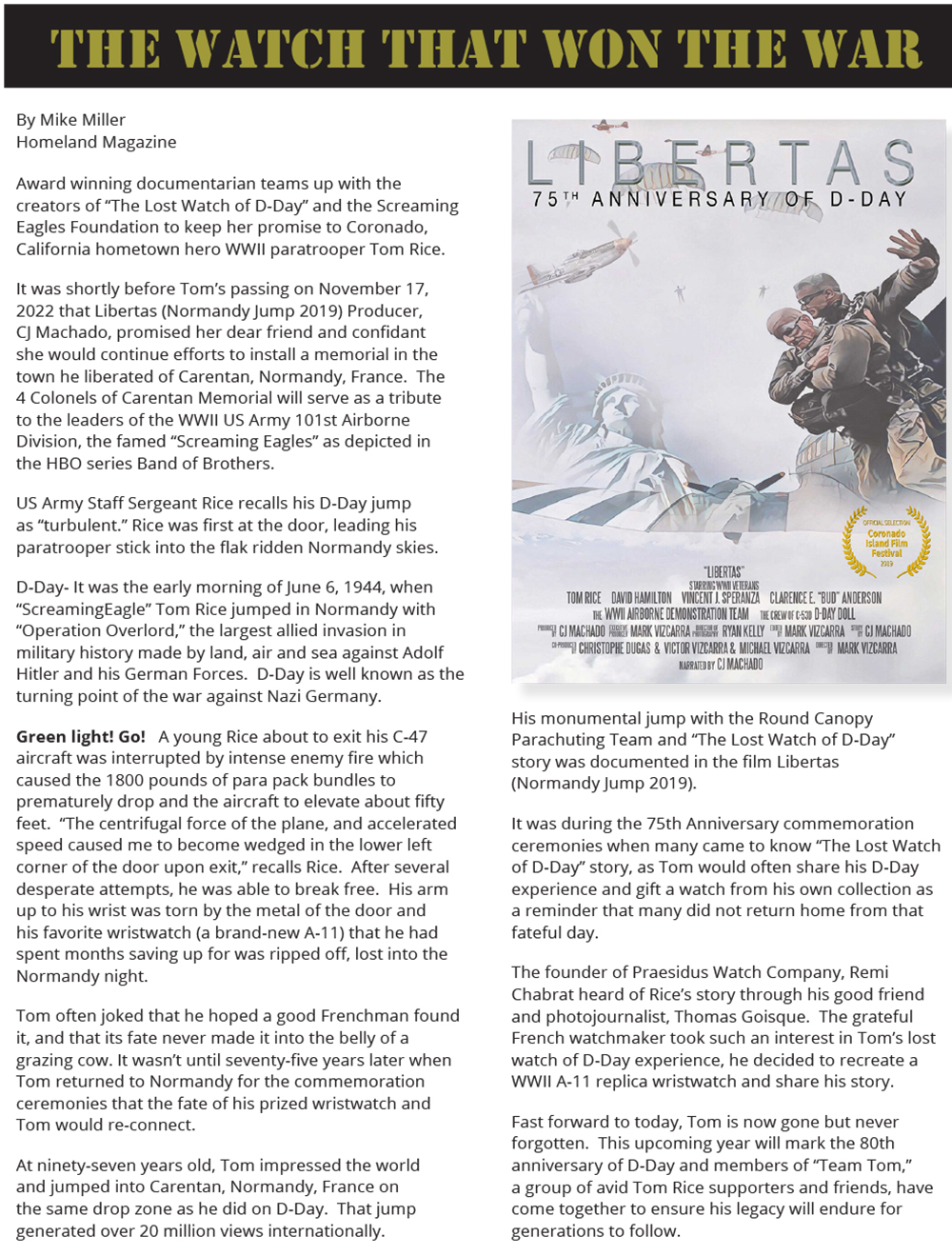This image features a highly detailed magazine article about D-Day, focusing on a significant element titled "The Watch That Won The War" by Mike Miller, published in Homeland Magazine. The article is divided into two columns of black text on a white background, with a prominent black banner at the top containing yellowish-gold text. Just below the banner sits a collage-like image that resembles a movie poster for "Libertas: 75th Anniversary of D-Day," featuring paratroopers, airplanes, and the Statue of Liberty.

The article highlights an award-winning documentary in collaboration with the creators of "The Lost Watch of D-Day" and the Screaming Eagles Foundation. The narrative centers around World War II paratrooper Tom Rice, a hometown hero from Coronado, California. The layout includes detailed text paragraphs on the left and a mix of text and images on the right, which features the visual elements mentioned. Colors in the image include grays, whites, light blues, tan, beige, and gold. The setting suggests a feature spread within a magazine.